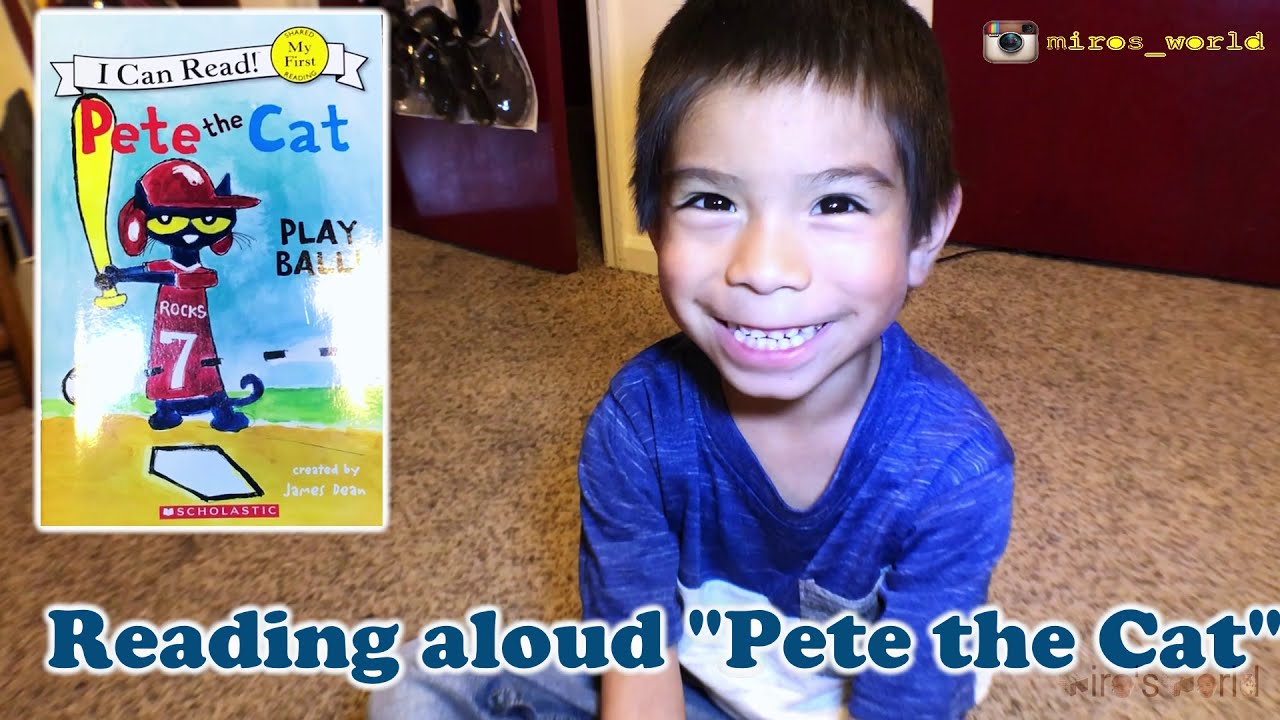The image features a joyous young Asian boy with medium-length brown hair and very dark eyes, his wide, teeth-baring smile causing his eyes to crinkle at the corners. He is seated cross-legged on a brown speckled carpet, looking up at the camera. He is wearing a medium blue shirt and light blue jeans. In the background, there's a maroon wall and door, alongside portions of a white wall.

On the left side of the image, a rectangular panel resembling a book cover is superimposed. The book cover reads "Pete the Cat" with "Pete" in red and "Cat" in blue. The title also includes "I Can Read" and "Play Ball." The cover depicts a black cat named Pete, with large yellow eyes, dressed in a red baseball uniform, holding a yellow bat, and standing at home plate, ready to bat. At the bottom of the image, the text "Reading Aloud Pete the Cat" is displayed, bordered in white. Additionally, the bottom right of the book cover notes it is created by James Dean and published by Scholastic.